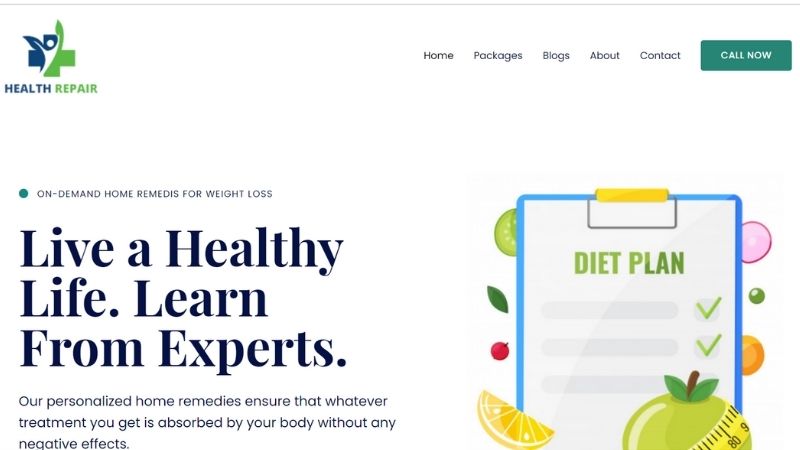The website for Health Repair prominently features a dynamic logo of a person with their arms raised above their head, resembling the lively, wavy figures often seen at car dealerships. The figure is colored in harmonious shades of blue and green, set against a similarly colored medical cross backdrop. The website's top navigation bar includes tabs for "Home," "Packages," "Blogs," "About," and "Contact," as well as a "Call Now" button for immediate inquiries.

Directly beneath the navigation bar, a headline reads "On-Demand Health Remedies" (note: "Remedies" is misspelled without the second 'e'). The slogan beneath it encourages users to "Live a Healthy Life, Learn from Experts," emphasizing the promise of their personalized home remedies, which are properly spelled in this instance. These remedies are designed to be effectively absorbed by the body without any adverse effects.

To the right of this introductory text, there's an illustration of a white clipboard with blue trim, featuring a distinctive yellow clasp, and a silver clip holding a sheet of paper. The paper, titled "Diet Plan" in green, is organized into imaginary columns marked with green check marks. Surrounding the clipboard are various fruits, vegetables, and leafy greens, symbolizing healthy eating. The image is completed with a green apple encircled by a measuring tape, visually reinforcing the website's focus on weight loss and overall health improvement.